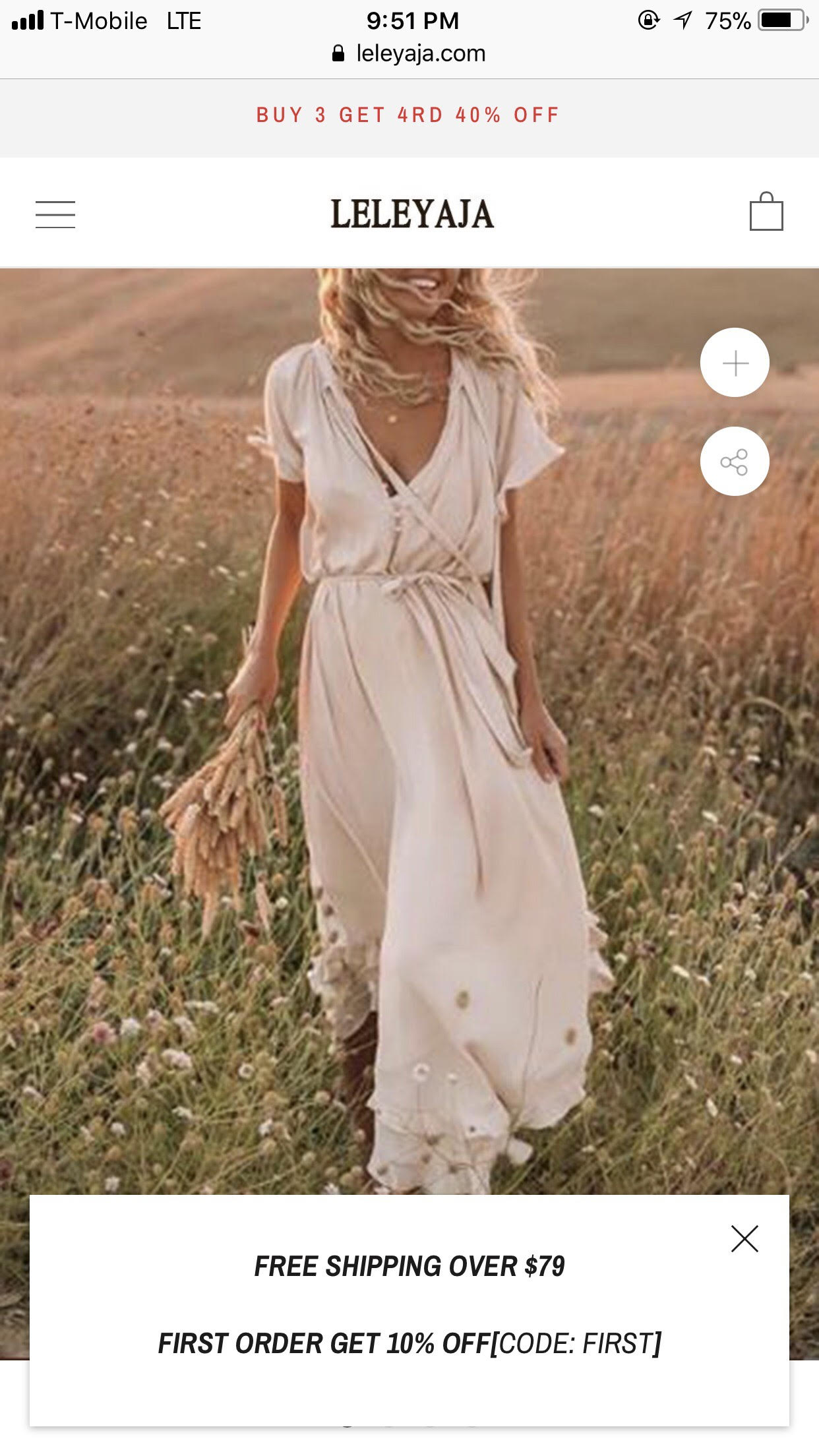The image captures a portrait screenshot of a mobile phone displaying the Leleyaja website at 9:51 PM, connected through T-Mobile with a 75% battery level. At the top of the screen, a promotional banner announces "Buy 3 Get 4th 40% Off." Below this banner, the interface showcases a menu icon on the left, the brand name "Leleyaja" prominently centered, and a shopping bag symbol on the right.

Dominating the screen is a large, striking photograph of a woman standing in the middle of a field filled with plants adorned with small white flowers. She is wearing a loose-fitting ivory maxi dress that flows gracefully in the wind. The dress has a loose collar that cascades between her breasts, revealing her bare arms. She holds a bundle of cut wheat stalks and appears to be walking towards the viewer. Though the photo only shows her from the mouth down to her ankles, it is evident that she has dyed blonde hair and artificially whitened teeth. Her skin is fair with a sun-kissed tan.

Below the photograph, promotional texts highlight two offers: "Free Shipping Over $79" and "First Order Get 10% Off."